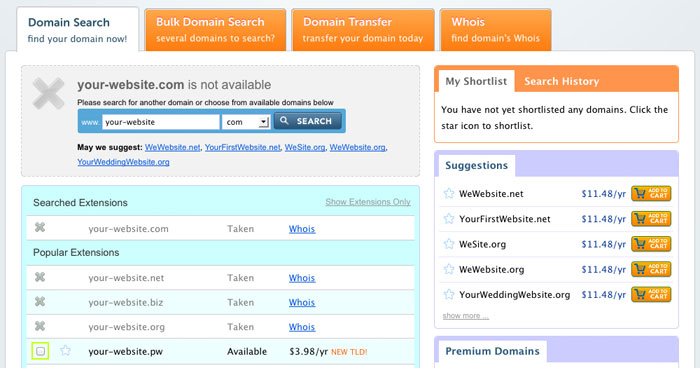The image depicts a domain search interface. At the top, there are four tabs with an orange background and white text, except for the selected tab, which is labeled "Domain Search - Find your domain now." This active tab has a white background and aqua blue font. Below this, a grayish box indicates that "your-website.com" is not available, suggesting that the user searched for this specific domain. 

At the bottom of the image, the interface is divided into two sections. The left section is designated for conducting searches, while the right section offers alternative domain suggestions along with their prices, which seem to be approximately $11.40 per year.